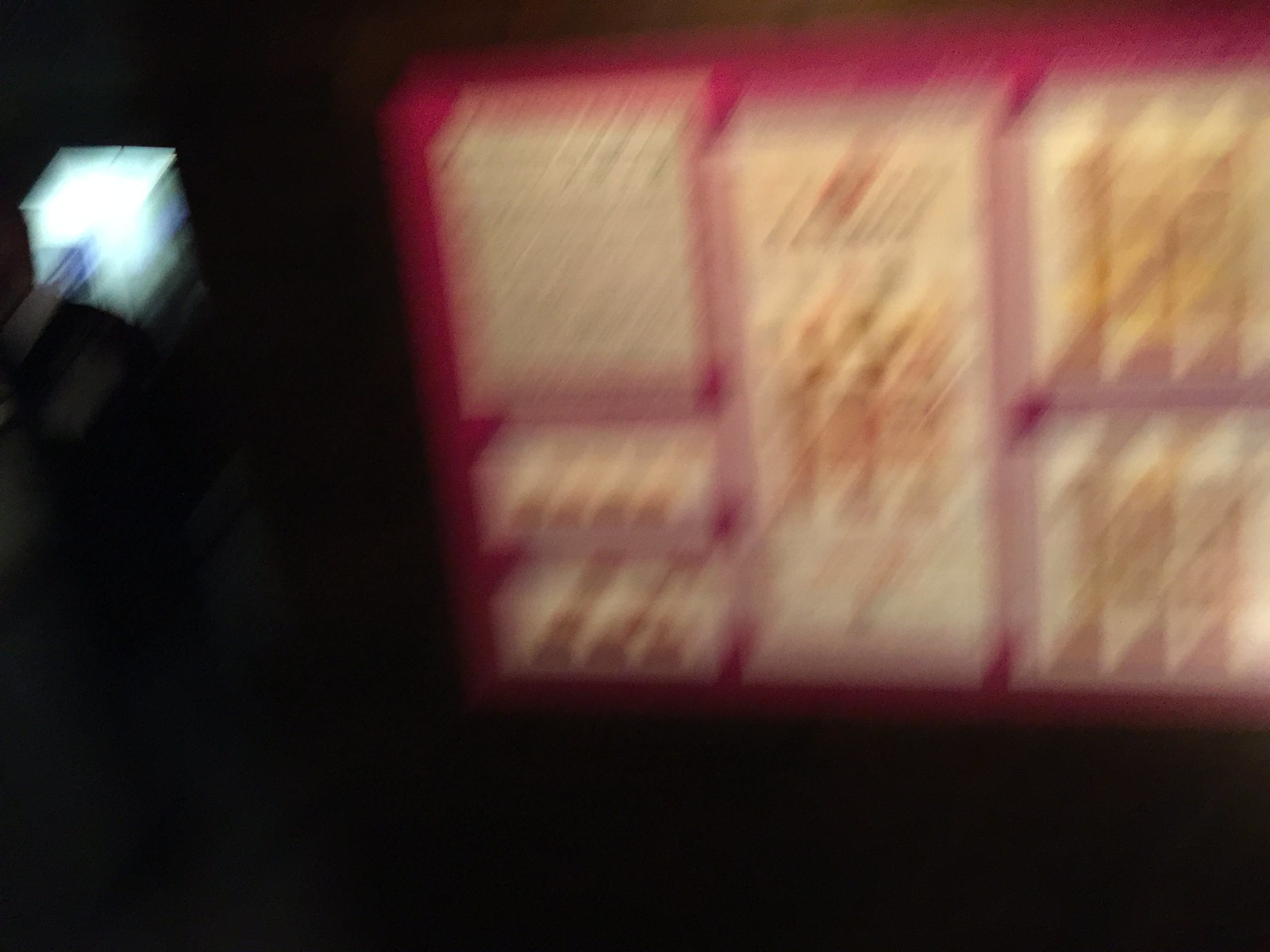The image depicts a blurry sign that appears to be some kind of menu, possibly belonging to a fast-food establishment. The setting is ambiguous, as it could be either an indoor or an outdoor location, but it is notably dark around the sign. The menu itself has a red border that segments different sections. Despite the blurriness, some items resembling burgers can be discerned, characterized by their brownish or yellowish hues. The background of the menu panels is a whitish or off-white color, standing out against the dark ambient surroundings. In the top-left corner of the image, there's a prominent, bright white light with a square shape, further adding to the contrast in lighting within the frame.